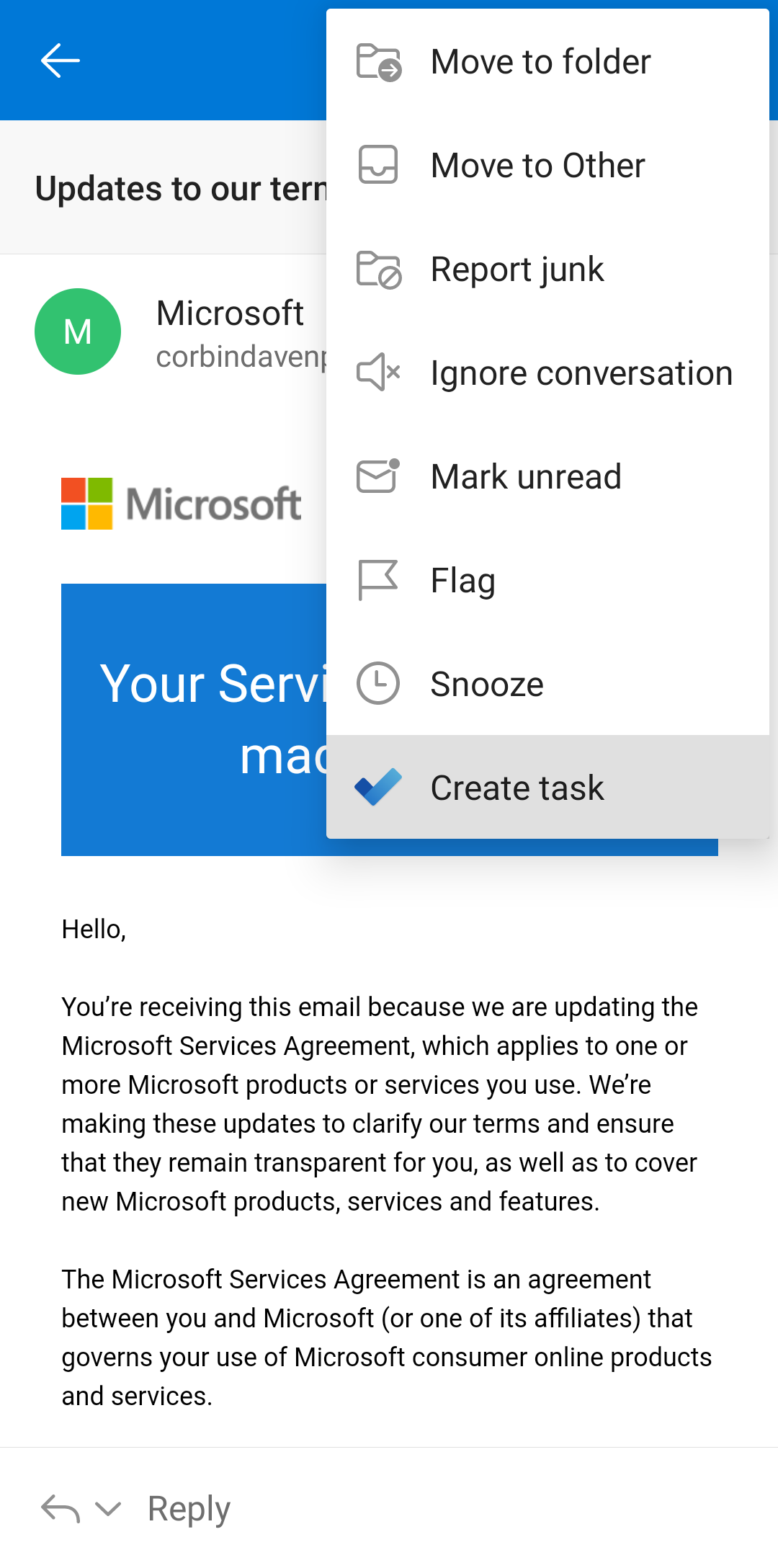This screenshot captures an email interface on a mobile phone. The screenshot is vertically elongated, indicating it's taken from a phone. On the top right corner, there's a pop-up menu offering options such as "Move to folder," "Move to other," "Report junk," "Ignore conversation," "Mark as unread," "Flag," and "Snooze." Each option is accompanied by a small graphic symbol— for instance, "Ignore conversation" features a speaker icon with a small "X" next to it.

Due to the pop-up obscuring part of the screen, only a portion of the email is visible. You can see the sender's details: at the top, it says "Microsoft," and below it, the name "Corbin Davenport" is displayed. The sender's profile icon is a simple green circle with a white "M" in the center. Additionally, a Microsoft logo is present along with a blue square that partially reads "Your service" before being cut off by the pop-up menu. The screenshot therefore offers a glimpse into the email but much of the content is hidden by the options menu.